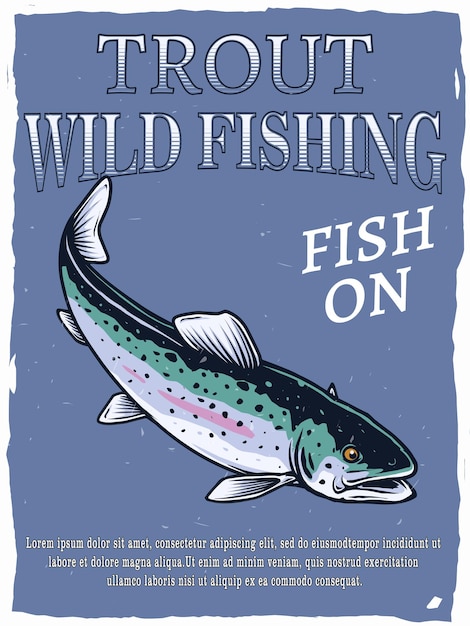The vertical rectangular poster features a periwinkle blue background with irregular and ragged edges, creating an uneven white border. Dominating the poster is a detailed drawing of a rainbow trout, characterized by its dark dorsal side, a greenish hue, a distinctive red and pink stripe through the middle, white underbelly, and gray fins. The fish’s eye is detailed with a black pupil surrounded by yellow, and its mouth is open, showcasing a lifelike portrayal. 

At the top of the poster, bold white letters, shaded blue at the bottom, proclaim "Trout Wild Fishing." Along the side, in plain white letters, the phrase "Fish On" can be seen. Below the image of the trout, there is some writing that appears to be in a foreign language, but the exact transcription is unclear. Overall, the poster, slightly taller than it is wide, appears old and weathered, suggesting it has been displayed for quite some time.